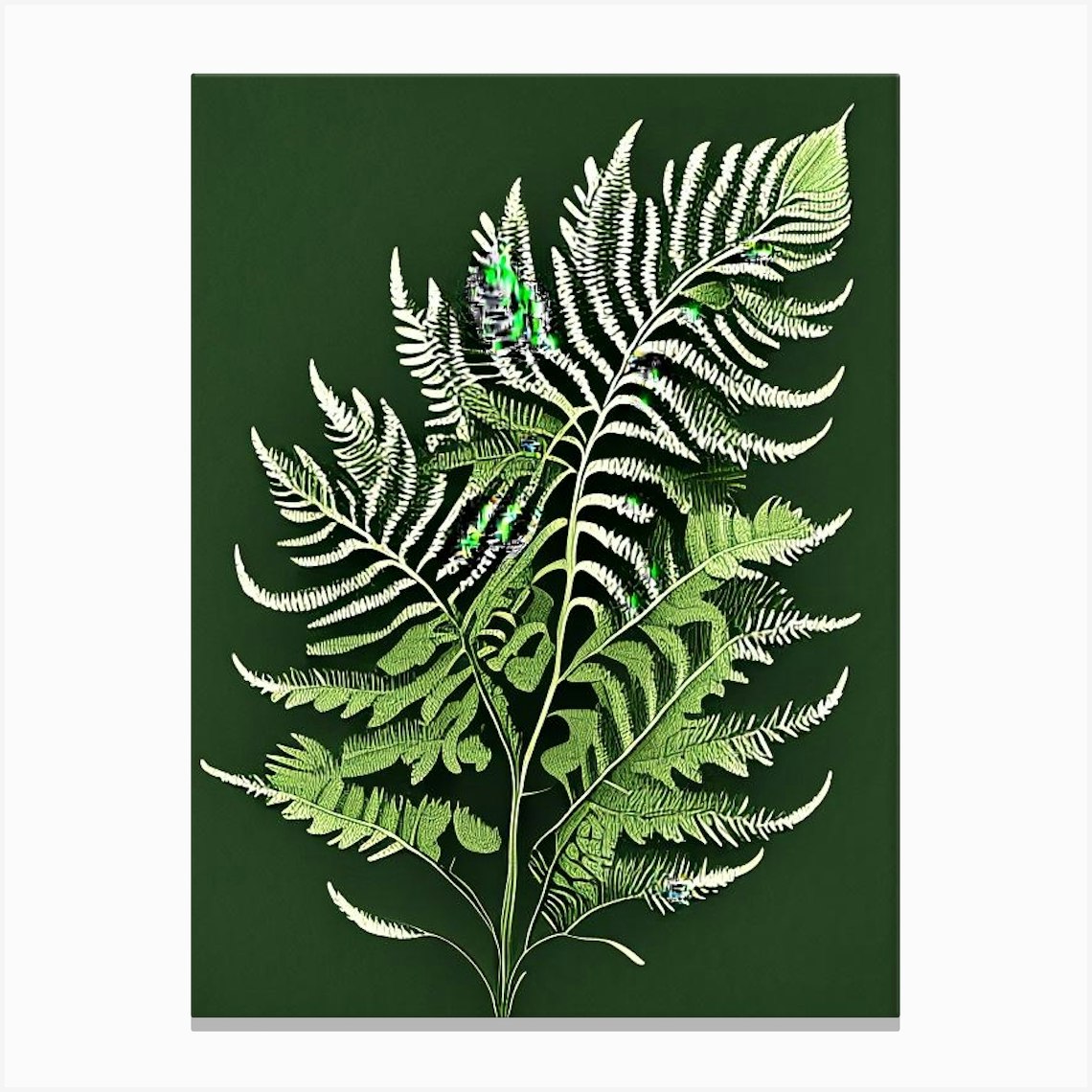This is a detailed color illustration of a fern leaf set against an olive green background. The fern is depicted with a range of shades, including light green, white, and lime green, making it very visually interesting. Some of the leaves are thin and white, while others are green and wavy, with bright neon green accents scattered throughout. The illustration is unique and blends various parts and patterns of different plants into a single cohesive image, creating a striking and non-traditional representation of a fern. The overall composition is vertical, enhancing its distinctive and eye-catching appearance.